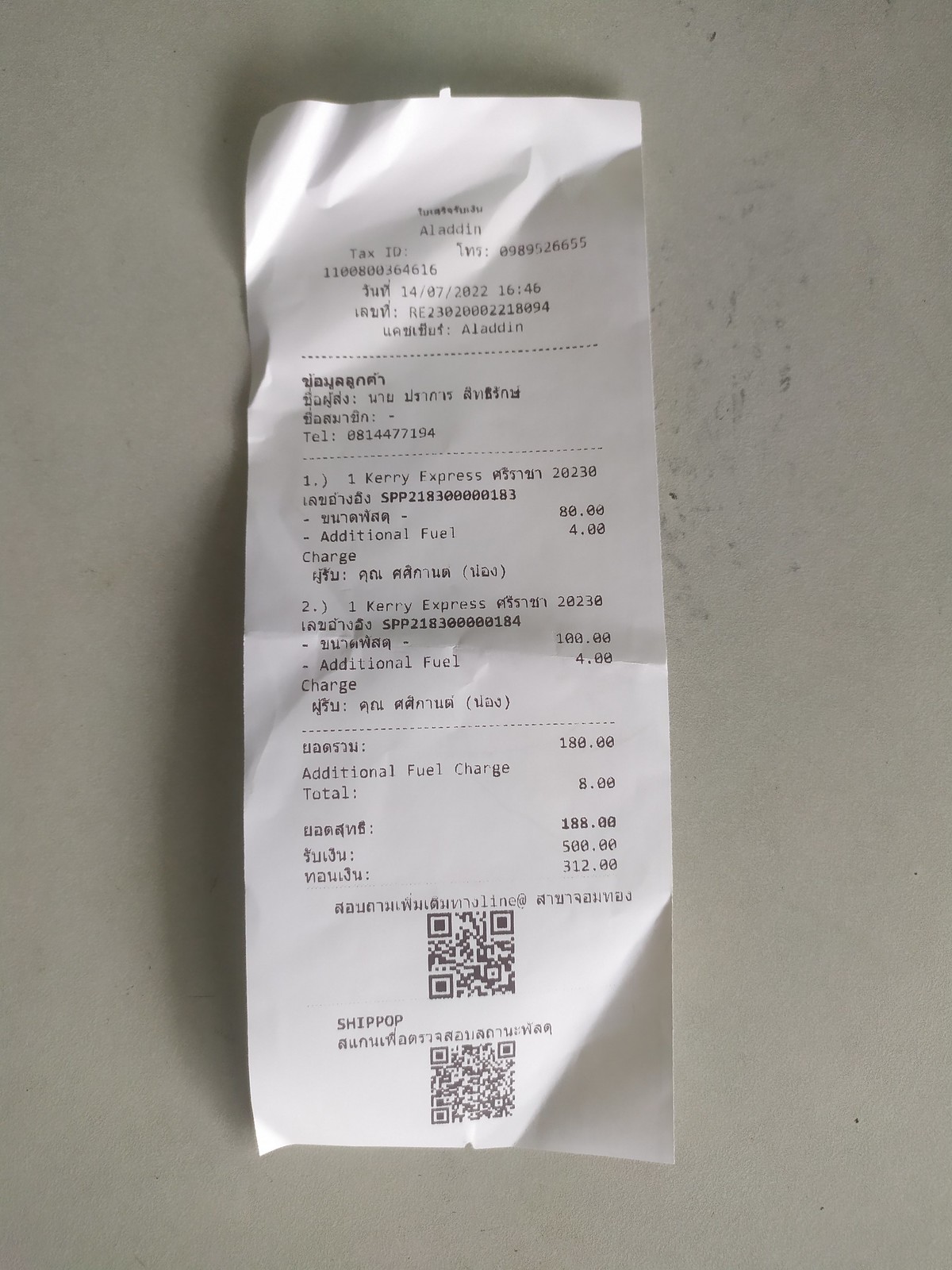The image displays a receipt laid out on a slightly dirty white countertop, which is dotted with some black specks. The receipt itself is rectangular in shape and slightly wrinkled at the top. Prominently displayed is the text "Aladdin Tax ID," which suggests the business or organization associated with the receipt. Much of the text on the receipt is in a foreign language, but there are several English terms and numerical values present. 

Specifically, the receipt mentions "Carry Express" and lists multiple charges:
- An initial charge of $80 with an additional fuel cost of $40.
- Another entry named "Carry Express 202 through 330" with a charge of $100 and an additional fuel cost of $4.
- An additional entry with a cost of $180 and an additional fuel charge totaling $8.

There are three separate numerical values listed: $188, $500, and $302. Finally, the receipt features two QR codes at the bottom.